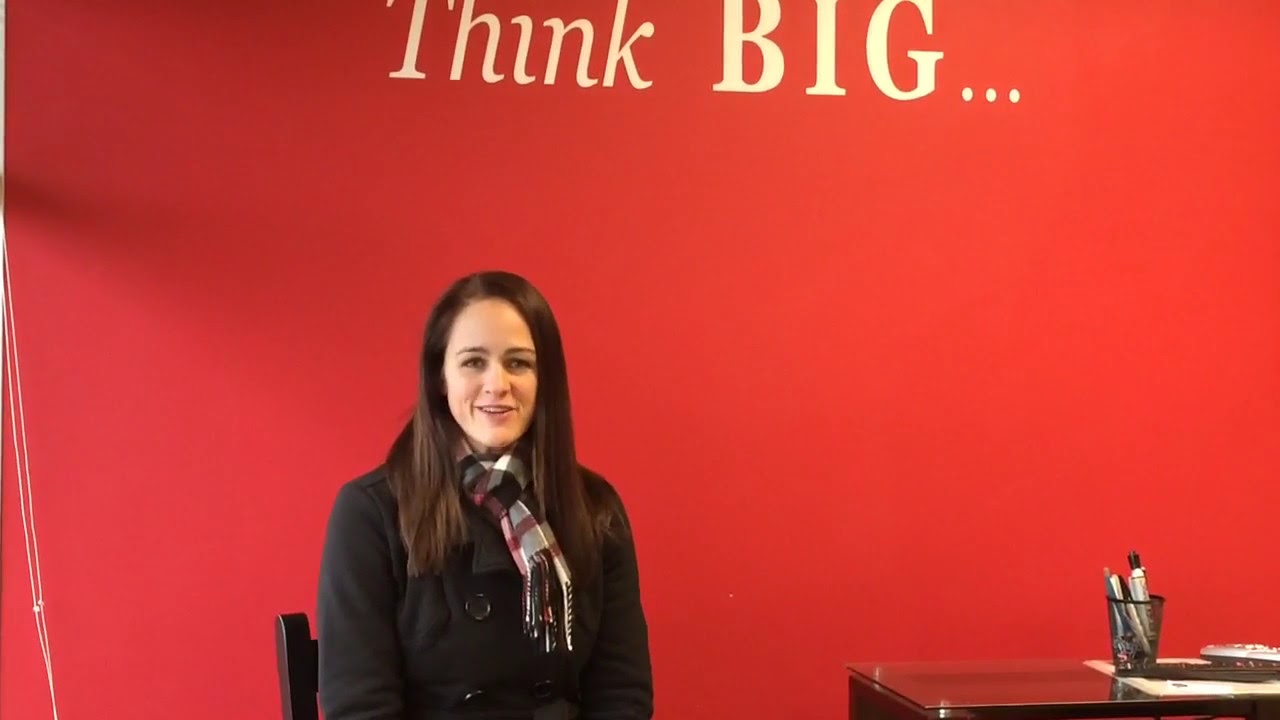In a photo set in a conference room or presentation space, a young white woman with shoulder-length dark brown hair wears a buttoned-up black jacket and a white, black, and gray plaid scarf accented with light red. She is seated in a brown chair, smiling and looking directly at the camera, possibly in mid-sentence. To her right, on a wooden desk, there is a black mesh container holding a magic marker and some pens, along with a silver and black TV remote control. In the background, a large red backdrop prominently displays the words "THINK BIG" in all caps and bold white font, with an ellipsis following "BIG". A white cord is also visible to her left, completing the scene.